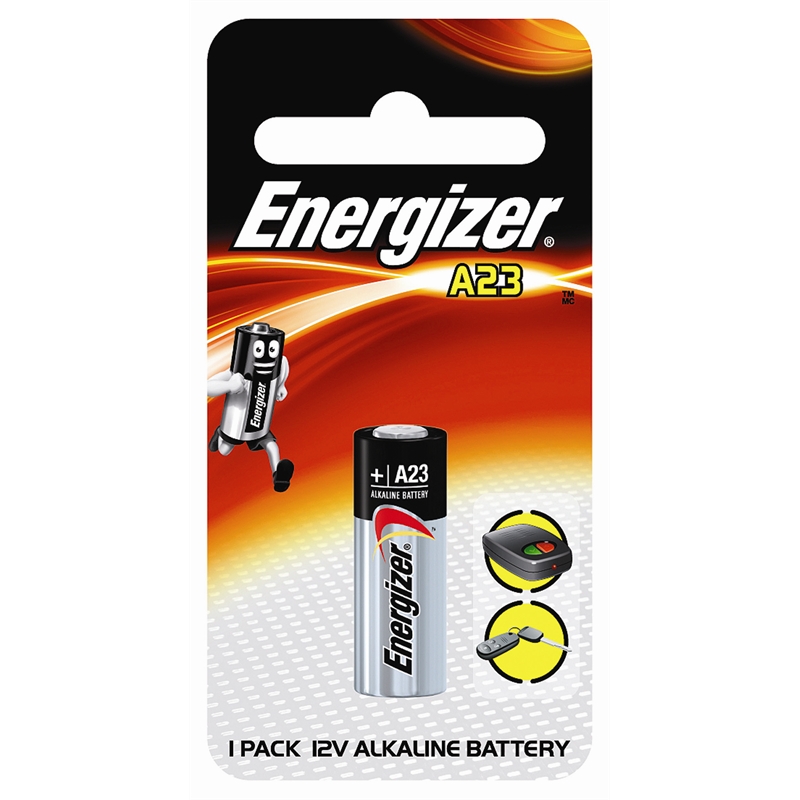This image showcases the retail packaging for an Energizer A23 12-volt alkaline battery. The packaging is designed with a black background complemented by a dark red-orange interface. Light streaks symbolizing electricity and energy course through the background, which also features a textured gray pattern for added depth. An identifiable Energizer mascot—a battery with a face, arms, and legs—is depicted running towards the viewer with a cheerful expression, emphasizing energy and approachability.

The front of the packaging prominently displays an image of the actual battery, clearly indicating that it is an alkaline type. It also includes visual icons illustrating two common applications: a key fob and a garage door opener. This particular pack contains a single battery.

Additional details, including various trademarks and copyright information related to Energizer’s imagery and slogans, are also present on the packaging. The top of the packaging features an opening designed for hanging on a store rack, ensuring visibility and accessibility for potential buyers.